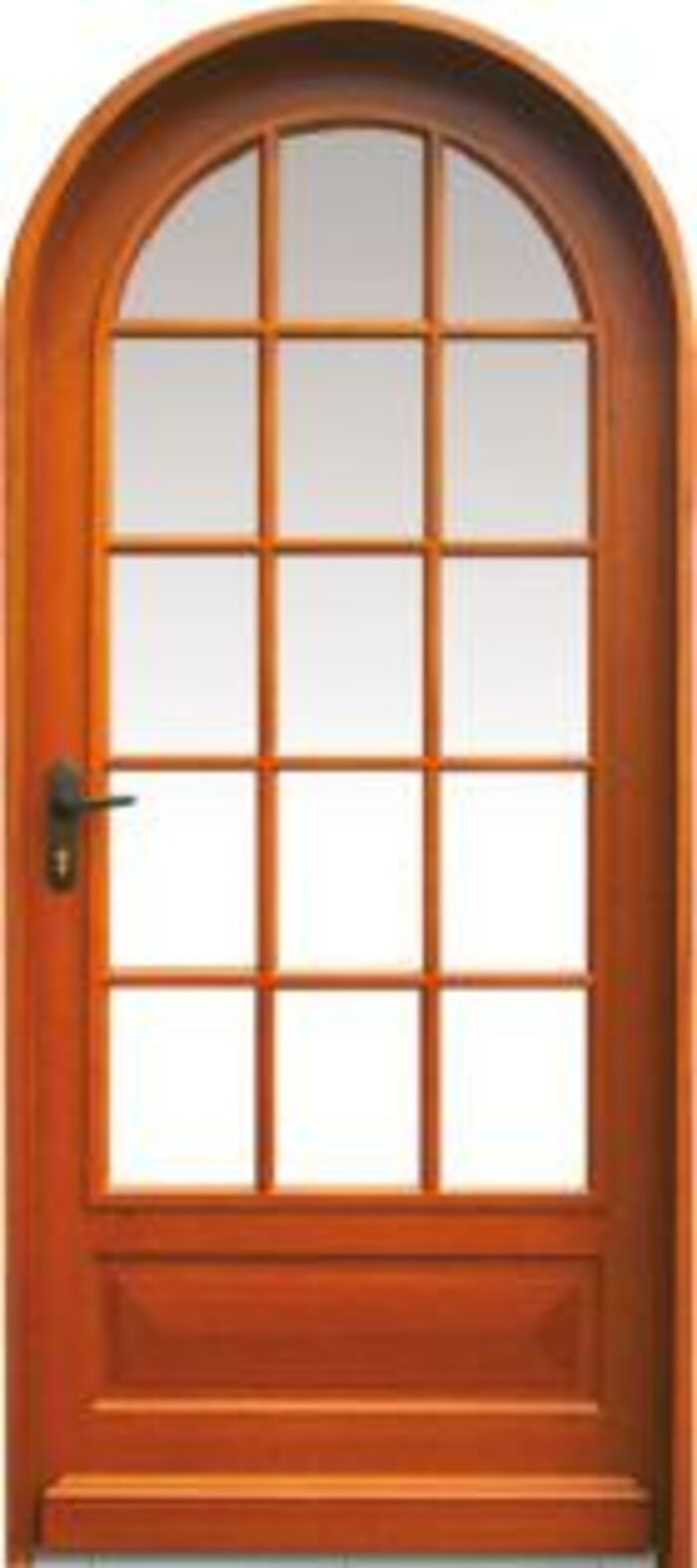This photograph showcases a wooden door with a distinct arched top and a flat, horizontal bottom. The door is composed of a rich, reddish wood, and features a large central window pane that spans approximately three-fourths of the door’s height, becoming a prominent design element. This window section is divided by thin wooden strips into a grid of fifteen panes: three horizontally aligned rows and five vertically aligned rows. Notably, the panes at the very top have a rounded shape to complement the door’s arched top. The remaining wood at the bottom quarter of the door is solid, providing a sturdier base.

The door also features a horizontally positioned metal pull handle located towards the center-left, characterized by its brownish-gold, possibly brass accents. Although slightly blurry, these accents are discernible at the base of the handle. Additionally, there is a subtle glimpse of the floor beneath, emphasizing the door’s realism and hinting at its functionality.